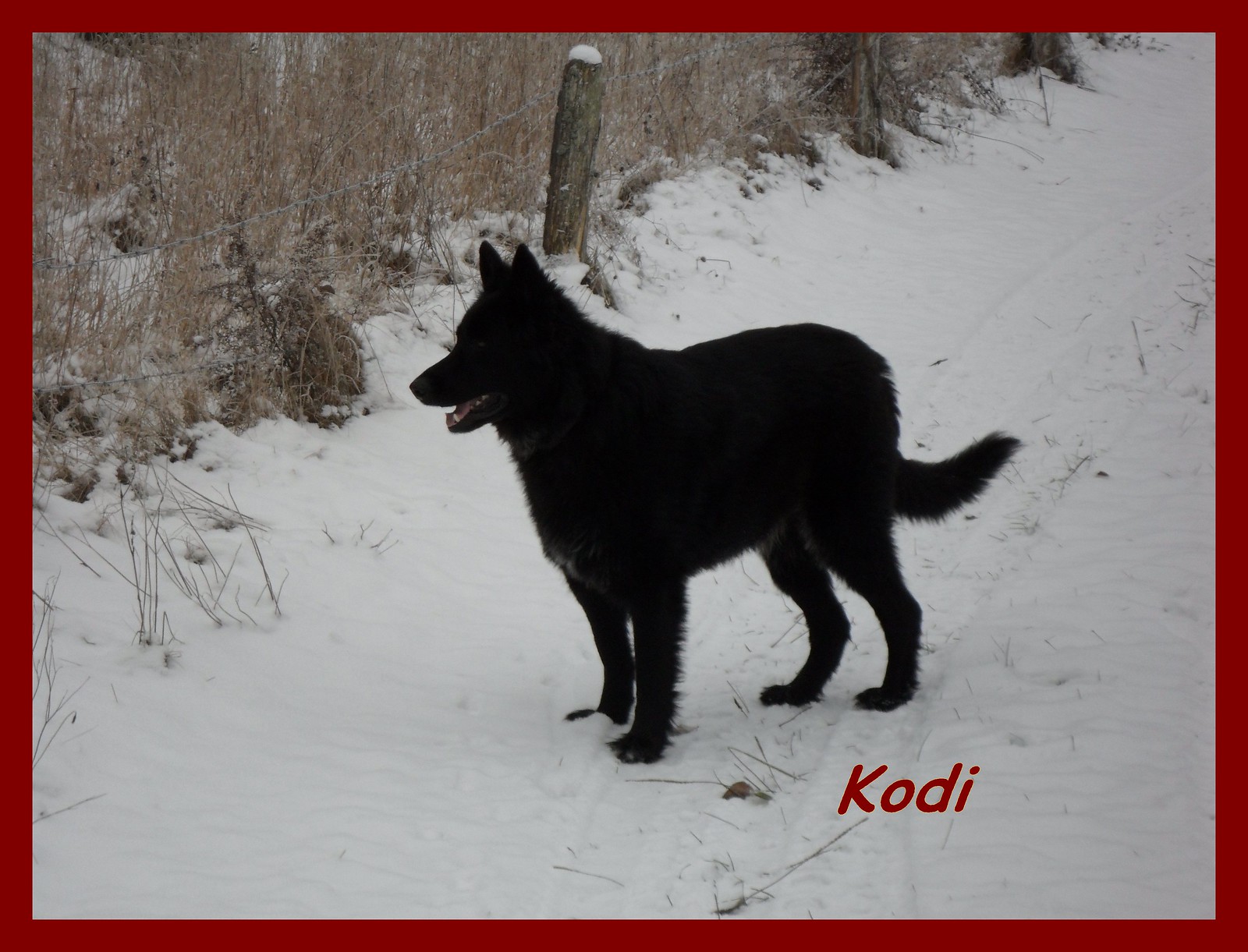This horizontally aligned rectangular photograph captures a large, black dog resembling a German Shepherd standing in the snow. The dog is furry, with a long tail, pointy ears, and an open mouth that reveals its pink tongue and canine teeth. Its eyes are almost invisible due to the darkness of its coat, and it slightly camouflages what appears to be a touch of white on its chest. The dog is looking to the left as though it's staring at something out of frame. In the lower right area of the image, the name "Cody," spelled "K-O-D-I," is printed in red. The background features tall, dead weeds or grass sticking through the snow, and to the left, a series of wood posts connected by chains forms a simple fence alongside what appears to be a natural trail or pathway. This entire image is framed by a red border, enhancing the vividness and focus on the scene.